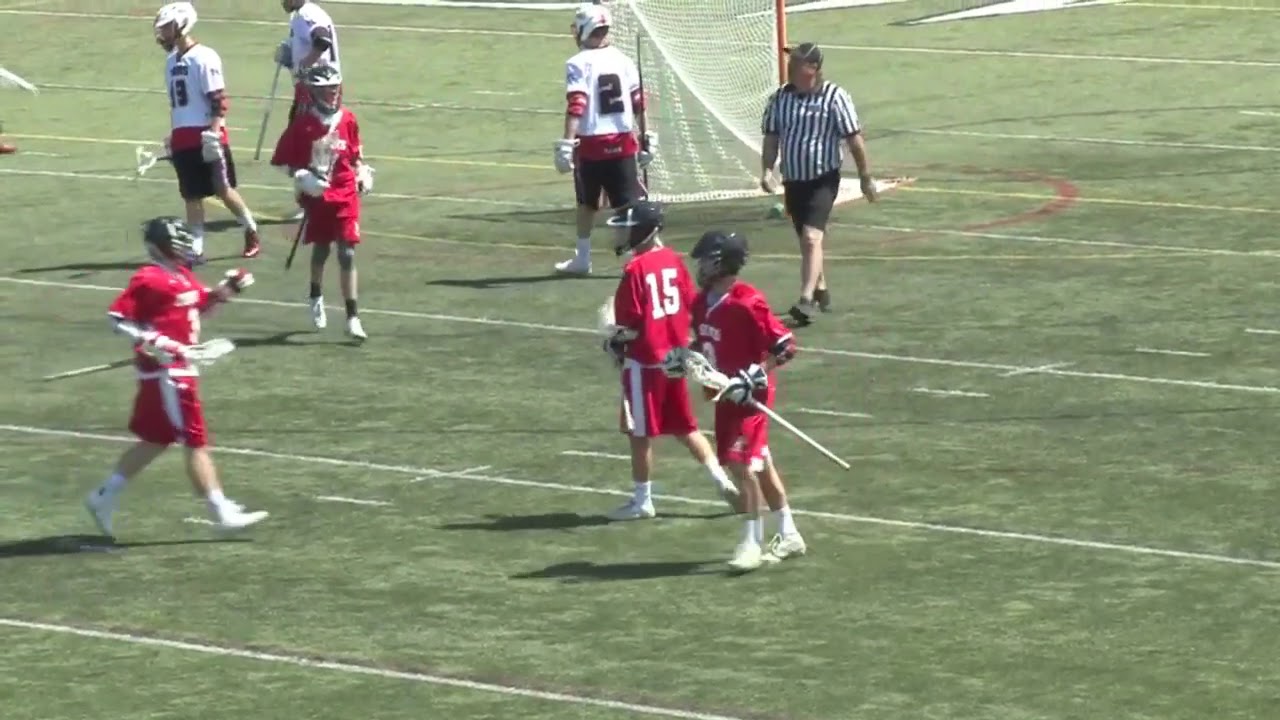The image depicts a lacrosse game being played on an AstroTurf field that appears to be a converted football field, as evidenced by the presence of football hash marks and lines. The teams are distinguishable by their uniforms: the red team, donning red jerseys with white numbers and red shorts with white stripes, is seen celebrating, likely having just scored a goal. In contrast, the white team, which sports white jerseys with black numbers, black shorts with red and white stripes, and white helmets, appears dejected with heads down, suggesting they conceded the goal. A peculiar sight includes the referee who is positioned in the background. He is wearing unusually short black shorts with a traditional black-and-white striped shirt and appears to be inattentively gazing away from the play, adding an odd detail with what looks like Crocs as his footwear. The field features clear white lines and a visible goal net framed by poles. The scene lacks active gameplay, as players from both teams seem to be standing around, possibly due to a recent goal or penalty. Sunlight casts shadows of the players, indicating a bright, sunny day.